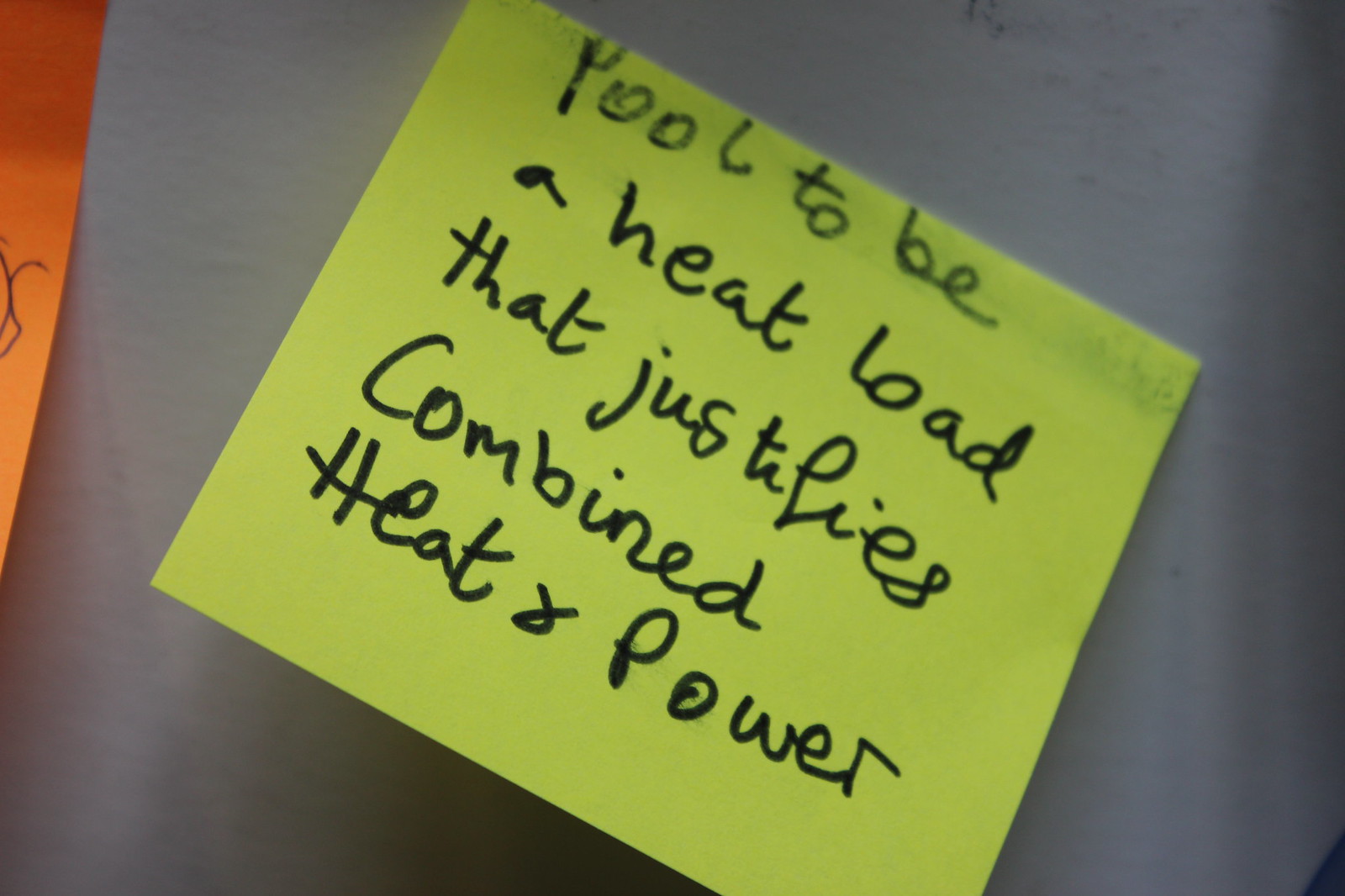In the image, the background is predominantly a whitish-gray wall, against which two post-it notes are affixed. The main post-it note is a fluorescent bright yellow, slightly tilted downward towards the bottom right. Written on this post-it in black marker are the words: "Pool to be a heat load that justifies combined heat and power." Notably, the phrase "Pool to be" appears to have been smudged, suggesting water damage, but the rest of the text remains clear. To the left side of the image, there's a partial view of a small orange post-it note with some text, though most of the writing on this orange note is obscured. The scene gives an impression of a cluttered workspace or brainstorming session with handwritten notes prominently displayed.